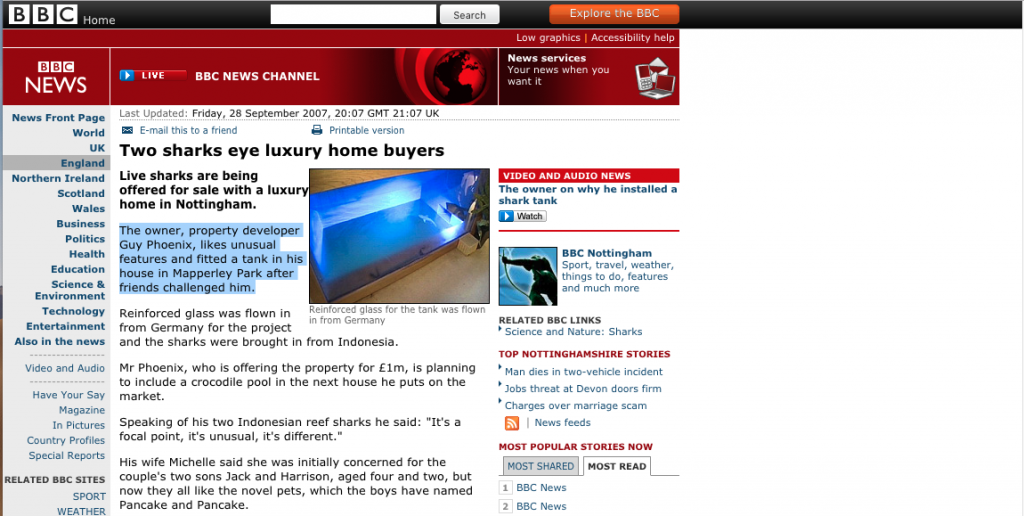The homepage of the BBC website features prominently displayed letters "BBC" in capital form, each within a white square, positioned at the top of the page. Below this, there's a search bar accompanied by a search button for easy navigation. A red rectangle labeled "Explore the BBC" with white text invites users to delve deeper. The page includes the BBC News logo, with the letters "BBC" in their distinctive white squares set against a red background, and "News" written in white next to it. 

An option to watch the **Live BBC News Channel** is available, alongside low graphics and accessibility help options for improved user experience. The news services section ensures that users can access the latest updates according to their preferences.

One of the highlighted articles features an intriguing headline about "Luxury Home Buyers," updated last on Friday 28 September 2007 at 20:07 GMT (21:07 UK time). There are convenient links to email the article to a friend and to print a version of it. The story narrates how live sharks are being offered for sale with a luxury home, an eccentric highlight chosen by property developer Guy Phoenix known for his taste in unusual features; one of which is a massive tank within the house.

Additionally, links for map and early parts in a PPR are noted within the details provided.